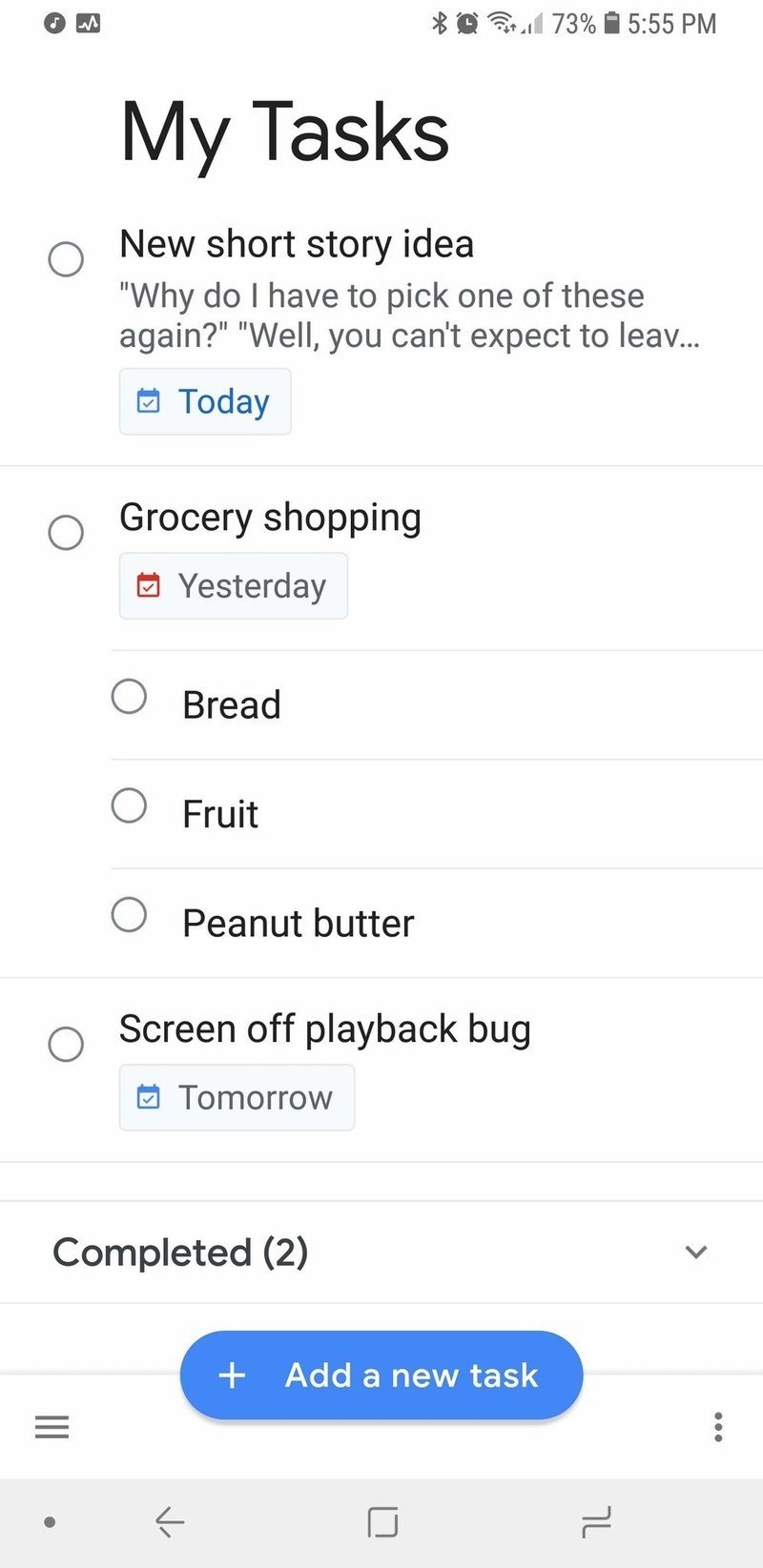The image displays a screenshot of a "My Tasks" page. At the top center of the page, there is a large black font with "My Tasks" written in it, with both "M" and "T" capitalized. Below this header, the tasks are listed:

1. A round circle indicative of a task marker is followed by the task "New short story idea." Accompanying this task are two quotes: "Why do I have to pick one of these?" and "Well, you can't expect to leave..." which trails off with ellipses. This task is marked with "Today" in blue text.

2. A dividing line separates the next section. The subsequent task is marked by another round circle and reads "Grocery shopping." This task is accompanied by a red calendar icon with a checkmark and the word "Yesterday." Following this are three bullet points listing items to purchase: bread, fruit, and peanut butter.

3. Another dividing line leads to the next task marker, which notes "Screen off playback bug." This task features a blue calendar icon with a blue checkmark, indicating the task is due "Tomorrow." Additionally, it mentions "Completed" with the number "(2)" in parentheses.

At the bottom of the list, a blue banner with white text contains a plus sign and the words "Add a new task."

This detailed interface captures a snapshot of a task management application's current task list, showing tasks scheduled for different days and providing a structured way to keep track of ongoing activities.